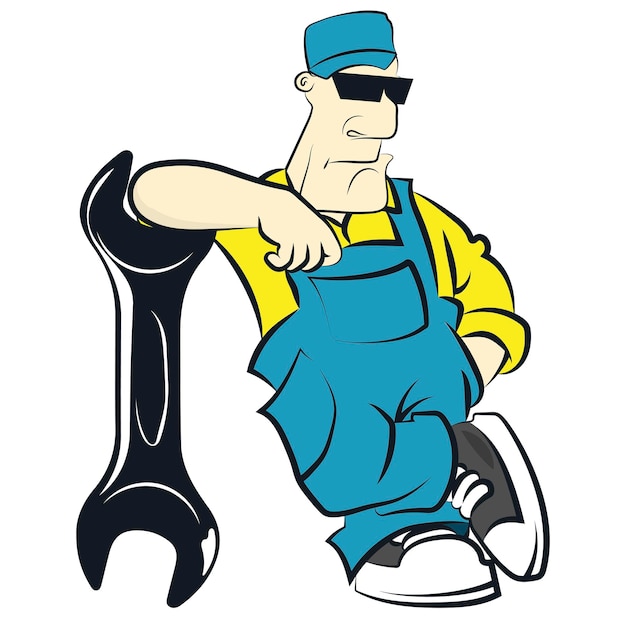The cartoon image depicts a mechanic-like man leaning nonchalantly on an enormously oversized black wrench that stands from the ground up to his shoulder. The man, with a pronounced square jaw and large nose, has Caucasian skin and small ears, and wears black sunglasses that obscure his eyes. He sports a blue painter's cap and blue overalls, paired with a long-sleeved yellow collared shirt with the sleeves rolled up just beneath his elbows. His left hand is casually tucked into the pocket of his overalls, while his right arm rests through the top part of the wrench, giving the impression that he’s leaning against it like a table. He has black and white sneakers with white laces and is posed with one leg crossed over the other. The backdrop of the image is completely white, emphasizing the vividness and exaggerated features typical of a cartoon style.